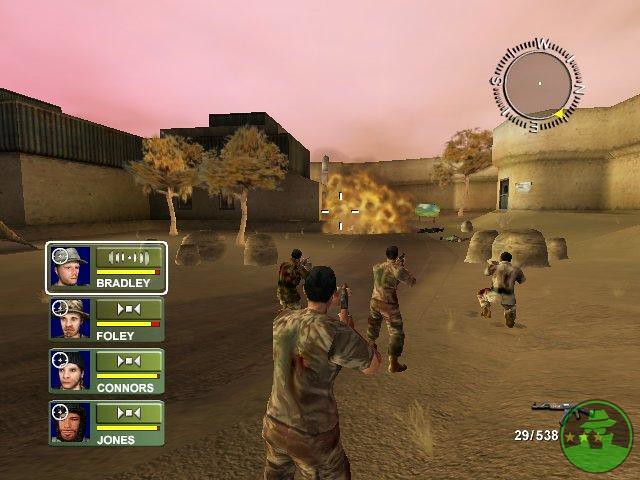The image depicts a detailed, colored screen capture from a wartime video game. In the foreground, four soldiers in camouflage uniforms, with short dark hair, are facing away from the viewer, aiming their guns forward as they traverse a sandy terrain. Their determined stance is directed towards a compound, partially enclosed by walls, where a dramatic explosion dominates the center of the background. Flanking the compound, a two-story brown building stands to the left, juxtaposed by another building on the right.

In the upper right corner of the screen, a compass points northeast, marked by a little yellow triangle. The compass clearly demarcates the cardinal directions: north on the right, east at the bottom, south on the left, and west at the top. Adjacent to the compass, the numbers "29-538" are displayed in white, accompanied by a circular logo. 

On the left side of the screen is a character scoreboard consisting of four rectangular images showcasing the digital faces of the soldiers. The top rectangle, outlined in white, displays the codename "Bradley." Below, in a similar layout but without the outline, are "Foley," "Connors," and "Jones," each accompanied by yellow lines with hints of red.

This pixelated, vividly detailed illustration showcases the intense and immersive environment typical of digital combat gaming.